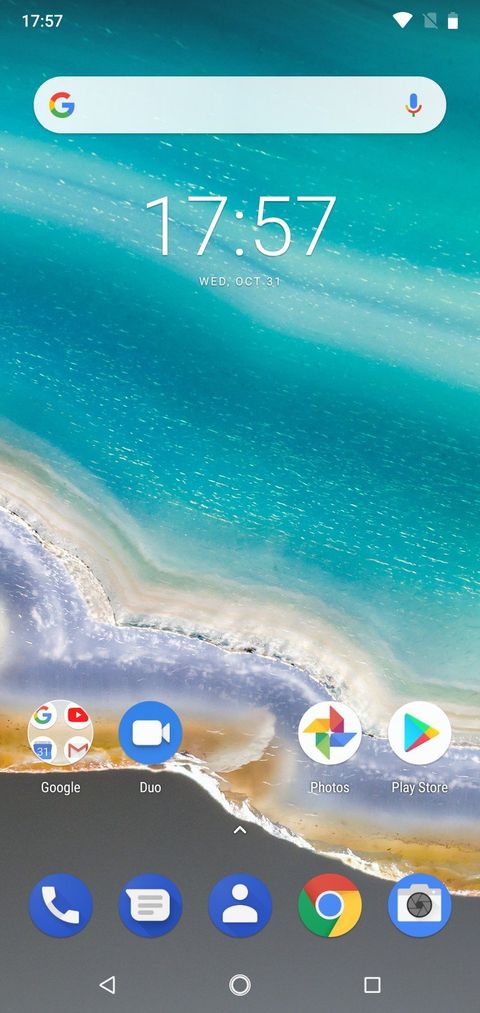The image depicts a cross-section of a geode, which vividly resembles a scenic beach at first glance. The geode features vivid layers with a variety of colors: a striking blue core, tan and blue concentric rings, and outer bands of slightly tan, brown, and gray. However, it's undeniably a rock formation, not an ocean view, as initially misleading.

Overlaying the geode imagery, a mobile phone's screen is captured:

- At the top left, the time reads "17:57" in white.
- A white Wi-Fi symbol, a grayed-out SD card slot icon, and a battery indicator at approximately 75% capacity are also visible.
- Below, a Google search bar with a microphone icon is present.

Mid-screen, there are icons for Google apps, including:
- Google in a circle
- YouTube
- Calendar
- Gmail
- Duo (displaying a camera icon)
- Photos (represented by a colored pinwheel)
- Google Play Store (with its trademark multi-colored triangle)

Towards the bottom left:
- A phone icon in white on a blue circle
- A chat icon in white on a blue circle
- A silhouette of a person in white, also on a blue circle
- Google Chrome's multicolored circle icon with a blue center dot
- A camera icon in gray with a blue circle

Beneath the app icons, the navigation bar includes:
- A back arrow
- A home button
- A tab button

Overall, the screen capture showcases both the detailed beauty of the geode and an organized display of app icons on an Android device.